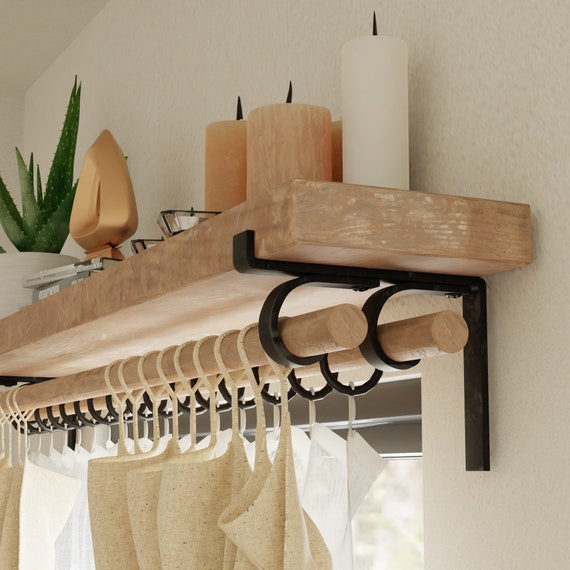The photograph shows an interior view of a cozy, well-lit room with natural light streaming through a window, partially obscured by a beige and white curtain. The wall is a neutral grayish-beige color, providing a soft background. Central to the image is a light brown wooden shelf, mounted at an angle with black brackets. These brackets not only hold up the shelf but also support two wooden curtain rods from which the curtain is suspended.

On the shelf, which spans across the middle of the image, there is a collection of decorative items. Starting from the left, there's a white pot containing a green cactus, a small, intriguing gold statue or trophy, followed by two white candles encased in a stylish black and glass holder. As you move further right, two peach-colored candles come into view, and finally, a long white candle with its top extending out of the frame is positioned near the edge of the shelf.

Below the shelf, the tan and white curtain hangs gracefully, partially covering the window beneath, while the black metal brackets provide a sturdy, industrial touch to the overall aesthetic of the room.